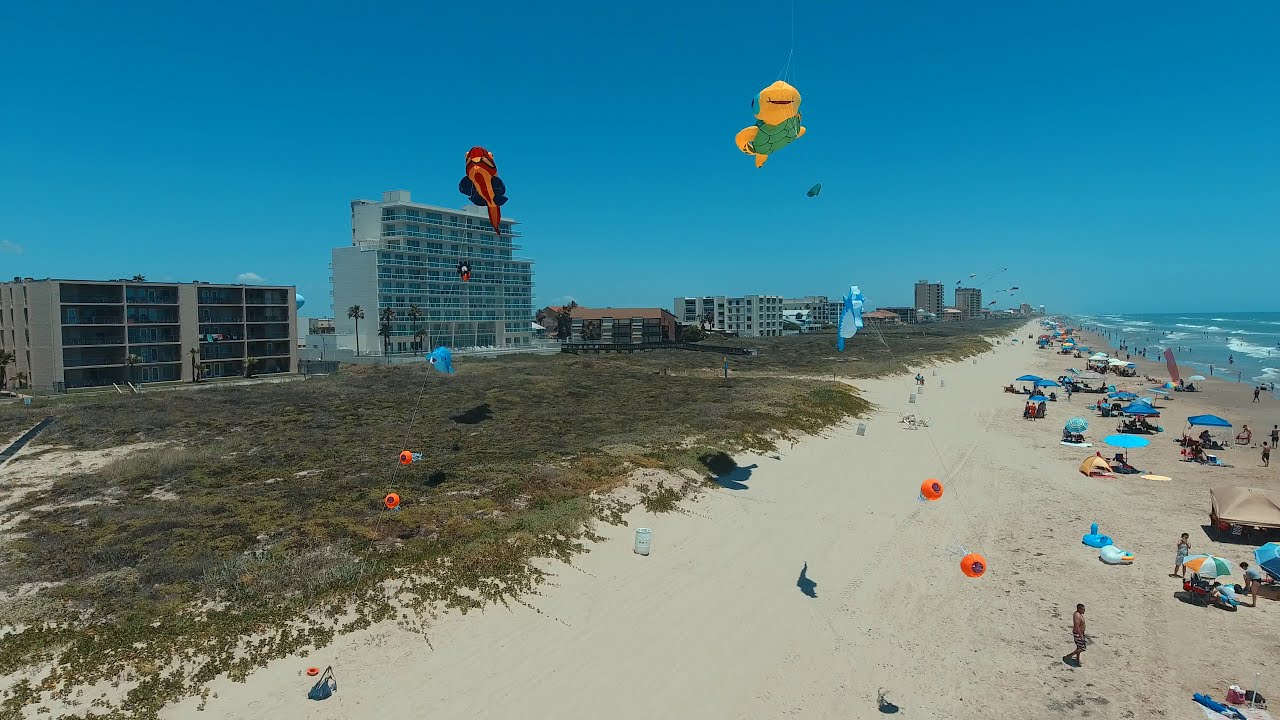The image captures a vibrant and bustling beach scene on a bright, sunny day. The long, light-colored sandy beach stretches across the right half of the photograph, populated with many people lounging under a mix of predominantly blue and some beige umbrellas. The left side of the image features a grassland area atop a sand dune, covered in a mix of dark brown and green foliage. This grassland extends towards the horizon where several multi-storied condo buildings stand tall. The tallest of these buildings is grey with numerous windows, while others have varied architectural features, such as a wide and flat four-story beige building with glass windows, and another slightly taller structure with a light blue and beige color scheme. The upper half of the image showcases a clear, deep cerulean blue sky filled with many kites, adding to the festive atmosphere of the beach. Notably, a kite resembling a red fish with black fins flies near the center-left, while another kite depicting a yellow turtle with a green belly soars to the right. In a small portion on the right edge of the image, the sparkling ocean water is just visible, completing the idyllic beach setting.